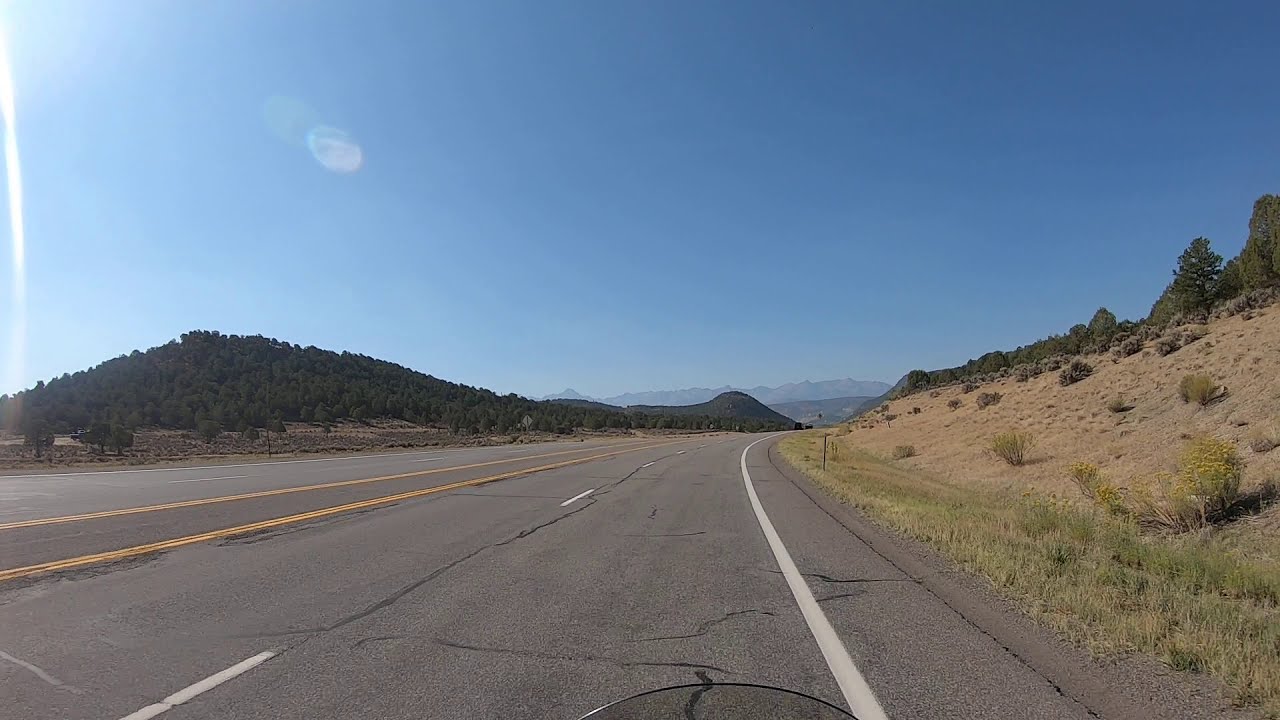This photograph captures a breathtaking outdoor landscape taken from the vantage point of a motorcycle rider, partially visible through the bike's curved windshield. It showcases a four-lane highway, composed of two lanes in each direction, made of gray concrete with evident cracks on the surface. The road is marked by white-painted lines on the right, white dotted lines in the center, and yellow divider lines on the left. There are no vehicles visible on the road, emphasizing its solitude.

To the left, the scene features a greenish mountain covered densely with dark green trees, giving way to hills that are similarly tree-laden. The right side of the road reveals more sparse vegetation, with mostly brown-yellow desert grass and hints of greenery. It transitions into rolling hills dotted with trees, and stretches into distant mountain ranges that frame the horizon. 

The atmosphere is impeccably clear under a bright, blue sky devoid of clouds. The sunlight is indirect, with rays emanating from the top-left corner of the image, casting a natural glow over the entire scene. The combination of the rural, hilly terrain with the open, sunlit sky creates a picturesque moment of serene beauty.